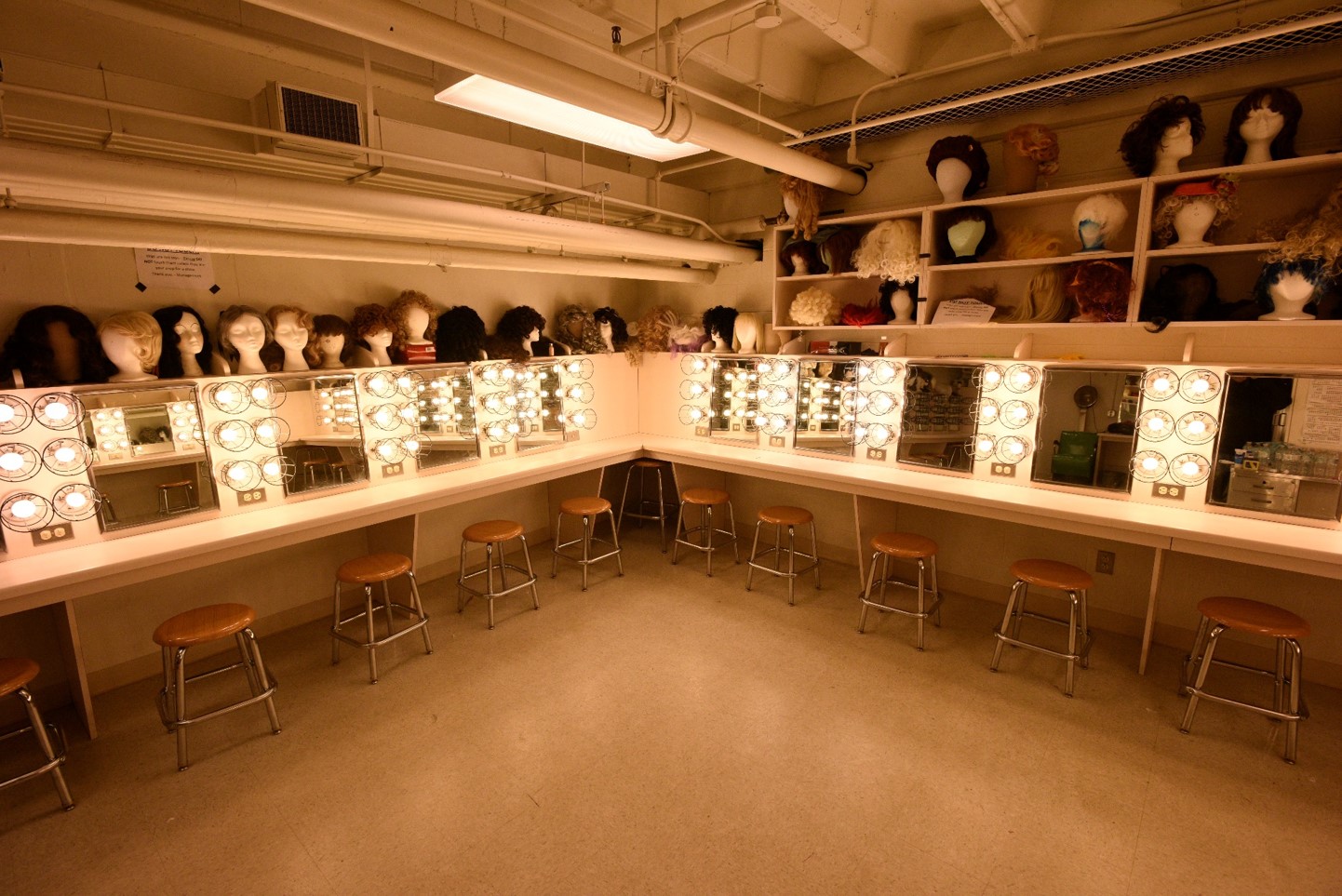The image depicts the inside of a dimly lit dressing room, likely situated in a basement given the visible maze of open pipes on the ceiling. The room, painted entirely in beige, exudes a warm yellow glow from the low overhead lighting. The focal point includes an L-shaped table fitted with multiple makeup stations, each equipped with a mirror surrounded by six lights, and a brown stool with stainless steel legs. Mannequin headstands populate the shelves and countertops, showcasing an array of colorful wigs – from brown and black to blonde. The room gives off a theatrical vibe, with its numerous vanities, mannequin heads, and costume wigs suggesting a preparation space for performers, perhaps in a theater or club setting.